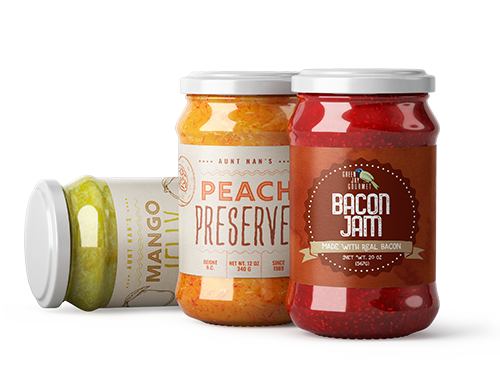This image is a detailed product shot showcasing three varieties of jams and preserves. On the left, a jar of mango jelly lies on its side, with a white label featuring the "Ant Man's" logo and smaller text. The clear glass container reveals a greenish substance inside. The jar in the middle is peach preserves, also from "Ant Man's," and it prominently displays the net weight of 12 ounces (340 grams) along with an establishment date from the 1900s on its white label. This jar contains an orange preserve that is visible through the glass. The jar on the right holds bacon jam made with real bacon, though from a different, unidentified company. It features a reddish-brown label and contains a red substance. All three jars are equipped with white painted metal twist-off lids, unifying the overall visual aesthetic.